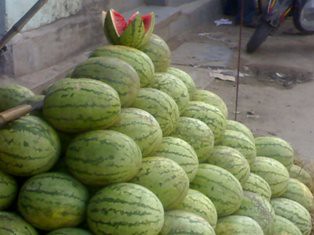In this close-up photo, a neatly stacked pile of approximately 25-30 watermelons rests on a light gray concrete surface. The stack, organized with precision, leans against a short wall that features a distinct pinkish stone border at its base. This wall transitions into a bluish hue towards the top and is accompanied by a small concrete path running alongside it. To the right, partially visible, is the tire and fender of a motorcycle adorned in red, yellow, and green. Among the watermelons, one has been split open in multiple segments, revealing its vibrant pink flesh and white rind, with small pieces scattered around. The scene captures a blend of textures and colors, from the light and dark green striped watermelons to the intricate details of the wall and the scattered pieces of the cut watermelon.